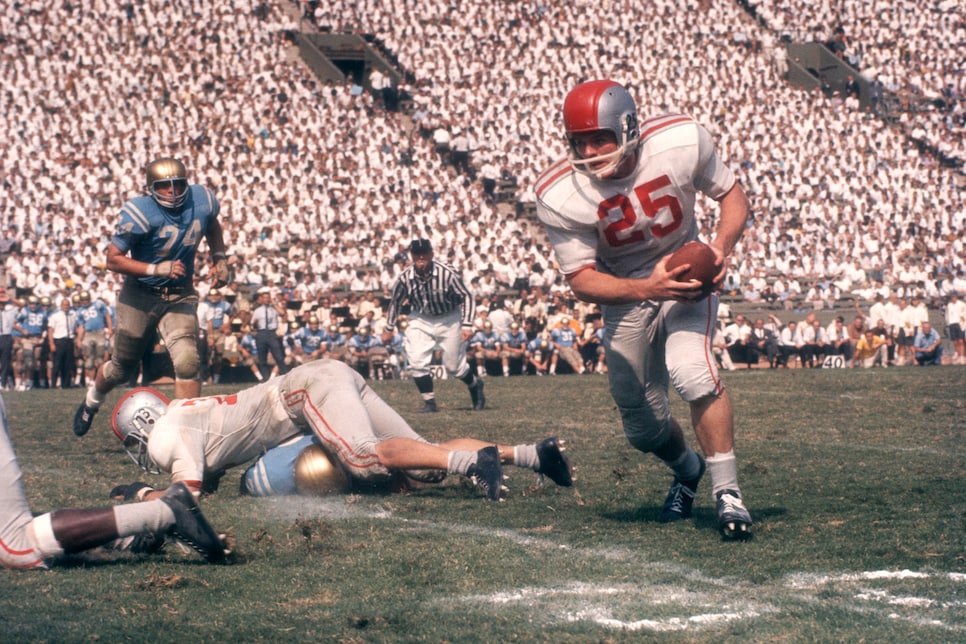This image captures an action-packed moment from what looks like a college or NFL football game, potentially from the 1970s. In the foreground on the right side, a football player wearing a silver and red helmet and a predominantly white and red uniform with the number 25 is running forward while clutching a brown football. Behind him, players from the opposing team, dressed in blue and white uniforms with gold helmets, are in pursuit. A dramatic scene unfolds beneath him, with one player from the blue team tackling another player to the ground. The scene is rife with motion and intensity, with several players visible in various stages of action. To the far right, a referee in a black and white striped uniform oversees the play. The background reveals a bustling stadium packed with thousands of spectators, all seemingly dressed in white, reflecting the high energy and collective excitement of the game. The stands are full to capacity, emphasizing the popularity and importance of this event. The atmosphere is electric, capturing the spirit of football in a bygone era.